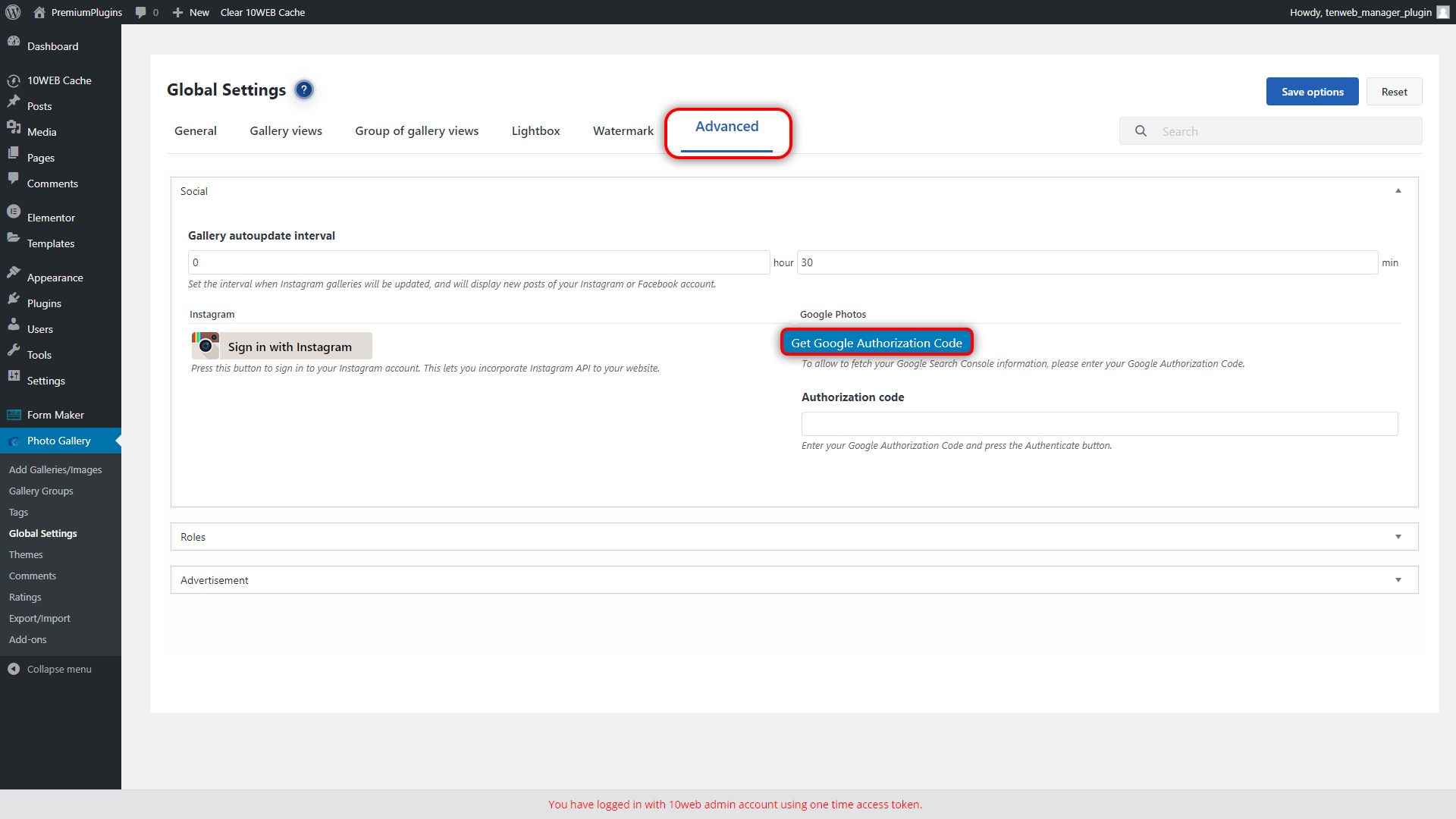This image is a detailed screenshot of a settings page for a photo gallery plugin within the WordPress dashboard. The WordPress interface is designed with a black sidebar on the left and a black top bar, both featuring light gray text. 

At the top left, we see the WordPress logo, a home icon, a small username display, and some additional text elements that are not fully legible. 

The black sidebar on the left contains navigational options such as:
- Dashboard
- Posts
- Media
- Pages
- Comments
- Templates
- Appearance
- Plugins
- Users
- Tools
- Settings

The main section of the screen is the plugin settings page with a light gray background. Dominating this area is a large white rectangle that contains all the plugin settings information. At the top of this section, there is a header labeled "Global Settings." Below this header, there is a submenu with tabs for different settings categories, including:
- General
- Gallery Views
- Group of Gallery Views
- Lightbox
- Watermark
- Advanced (This tab is highlighted in blue with an underline, indicating it is currently active.)

The user editing the image has added a red rectangle with rounded corners and a prominent shadow around the advanced settings tab.

In the upper right corner of the settings section, there are two buttons:
- "Save Options" (blue with white text)
- "Reset" (gray with black text)

Below these buttons are two input fields, initially set to zero and thirty, and options for connecting social media accounts:
- "Sign in with Instagram"
- "Google Photos"

Next to the Google Photos option is a blue button labeled "Get Google Authentication Code," also outlined in red by the user.

Further down are additional fields and configuration options, which are not detailed in this description.

At the very bottom, centered on a gray bar, is text in pink or red that appears to say, "You have logged in Admin," followed by some illegible text regarding a token.

Overall, the image captures a comprehensive view of a WordPress photo gallery plugin's settings interface, highlighting various configuration options available to the user.